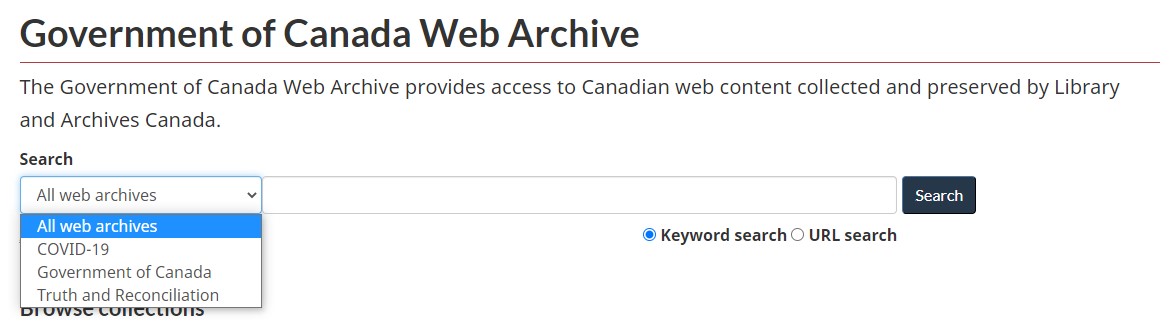This image is a screenshot of a webpage from the Government of Canada Web Archive. The layout is simple, with a clean white background and no borders. Dominating the upper left-hand corner, large text reads "Government of Canada Web Archive," beneath which is a thin purple horizontal line. Below this heading, an informative sentence states, "The Government of Canada Web Archive provides access to Canadian web content collected and preserved by Library and Archives Canada."

Further down the page, a search interface is presented. At the top of a pop-up box within this interface, the word "Search" is displayed, indicating the function of the dropdown menu below it. The dropdown menu lists four categories: "All Web Archives," "COVID-19," "Government of Canada," and "Truth and Reconciliation," with "All Web Archives" highlighted in blue.

Below the dropdown menu, partially visible beneath the pop-up box, the text reads "Browse Collections." Adjacent to this, on the right, lies a search bar with a dark grey search button. At the bottom-right corner of the search bar, two buttons are visible: "Keyword Search" and "URL Search." The "Keyword Search" button, marked by a blue dot, is currently highlighted.